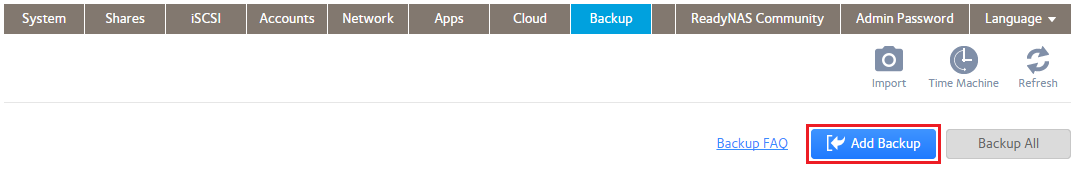**Descriptive Caption:**

The image displays the interface of a management system with a detailed menu bar located at the top. The menu bar features white text on a brown background and is divided into several segments. 

From left to right, the segments are labeled: "System," "Shares," "iSCSI" (with lowercase 'i' and uppercase 'SCSI'), "Accounts," "Network," "Apps," "Cloud," the selected "Backup" (highlighted with a blue background), "ReadyNAS Community" (with 'ReadyNAS' in camel case — 'Ready' in lowercase and 'NAS' in uppercase), "Admin Password," and the final segment "Language" which features a downward arrow indicating a pull-down menu for language selection.

Below the menu bar are three icon buttons: 
1. A camera icon labeled "Import"
2. A clock icon labeled "Time Machine"
3. An arrow circle icon labeled "Refresh."

Underneath these icons, the interface shows a "Backup FAQ," a highlighted blue button with a red border labeled "Add Backup," and another button labeled "Backup All."

The background of the page is simple, with no additional elements at the bottom. The overall design is clean and focused on the backup functionality of the management system.